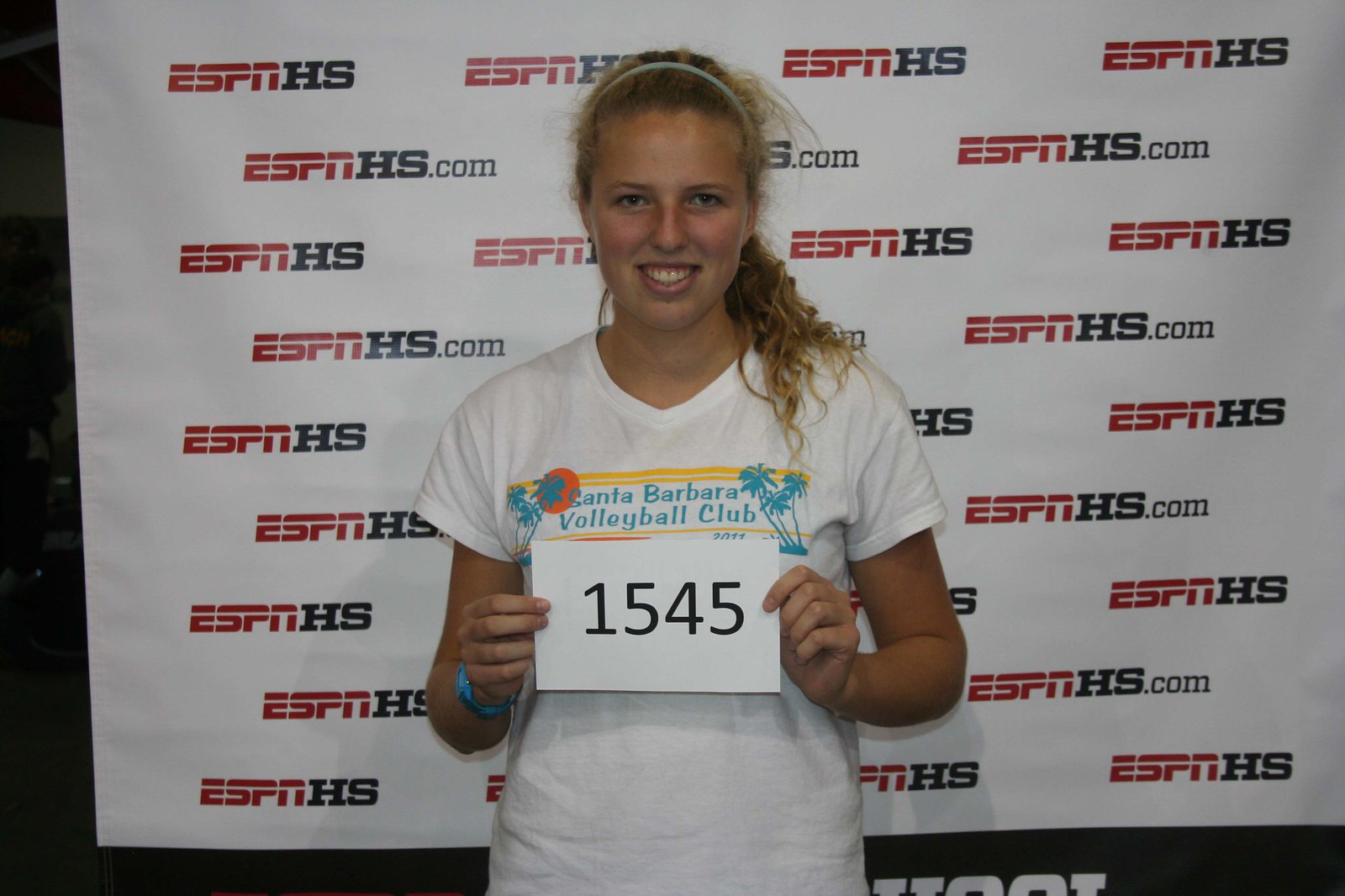A young woman with frazzled blonde hair pulled back by a thin headband stands in front of a large white banner repeatedly printed with "ESPN HS" in red and black. She gazes directly at the camera with a smile, revealing her top row of teeth. Dressed casually in a short-sleeved, v-neck white t-shirt adorned with pine trees on both sides of her chest and an orange sun on the right, she proudly displays the text "Santa Barbara Volleyball Club" emblazoned across her chest. Her arms are bent at the elbows, and she holds a white card with the number 1545 printed in black, close to her waist. The setting appears to be indoors, likely a promotional event or photo opportunity linked to ESPN's High School Sports coverage.